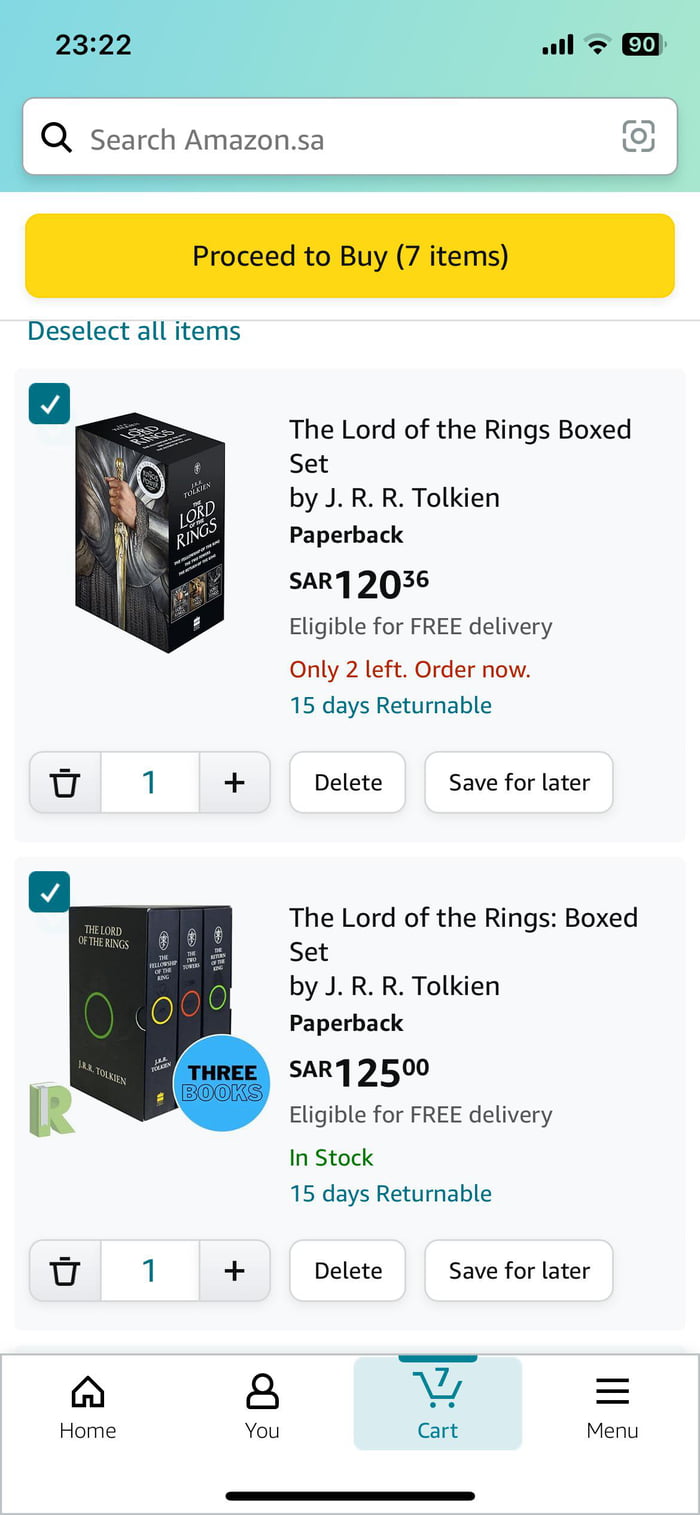This image is a screenshot from a smartphone displaying a shopping app in military time, specifically at 23:22. Starting from the upper right corner, the phone's status bar indicates a full four-bar signal strength, partial Wi-Fi reception with two full bars, and a battery level at 90%. Below, there is a white search bar labeled "Search Amazon."

Beneath the search bar, a prominent yellow rectangular button reads "Proceed to Buy" with a note that there are seven items in the cart. Following this, there is an option to "Deselect all items."

The shopping list includes two similar items, both checked:

1. **The Lord of the Rings Box Set by J.R.R. Tolkien**
   - Format: Paperback
   - Price: SAR 120.36
   - Additional Info: Eligible for free delivery, only two left in stock, and 15 days returnable.
   - Accompanying Image: Shows the book set.

2. **The Lord of the Rings Box Set (3 Books) by J.R.R. Tolkien**
   - Format: Paperback
   - Price: SAR 125.36
   - Additional Info: Eligible for free delivery, only two left in stock. No mention of returnability.
   - Accompanying Image: Shows the book set.

At the bottom of the screenshot, there are four navigation icons, likely part of the app's interface for easy access to different sections of the app.